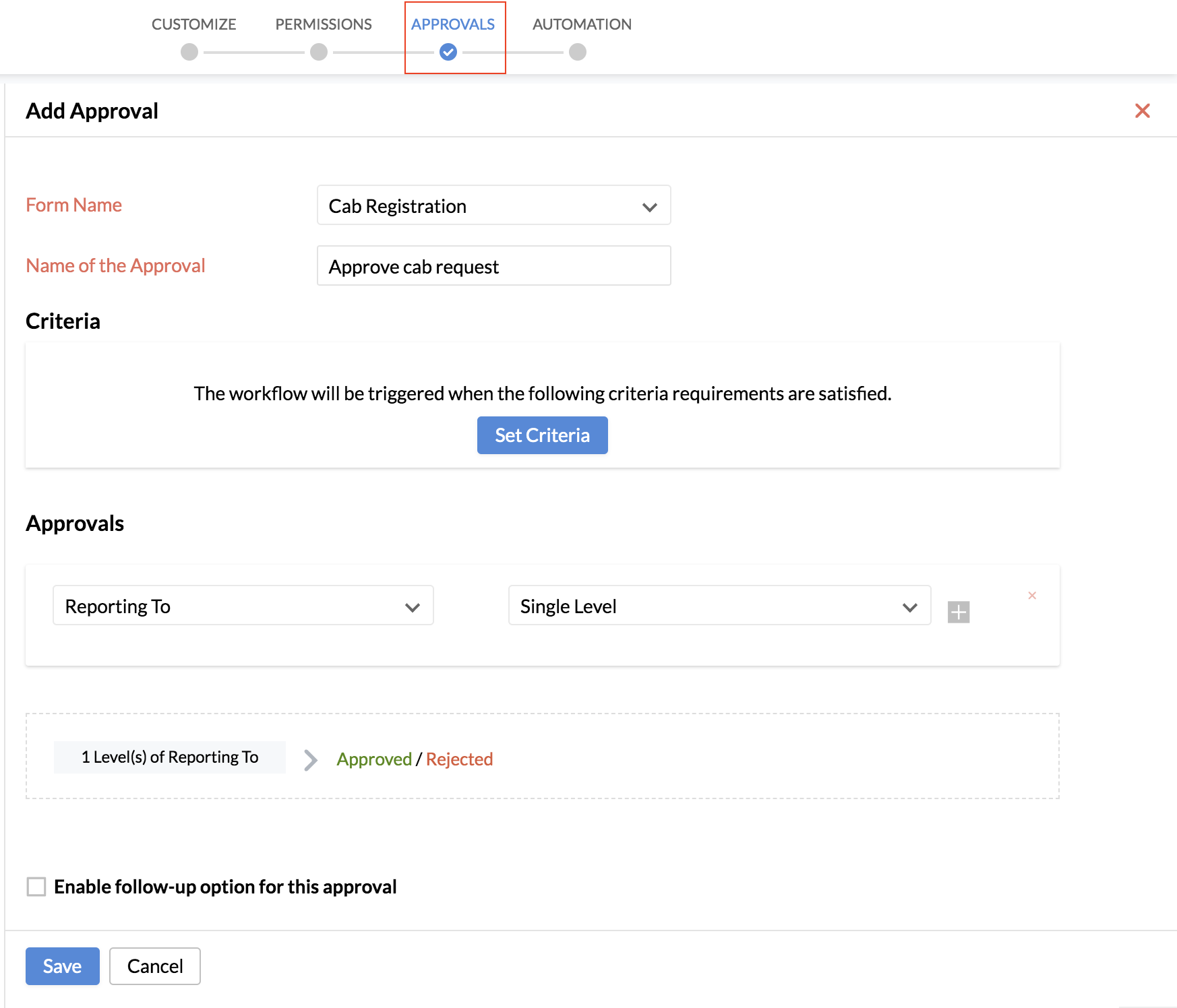The image depicts a detailed user interface for customizing workflow approvals. At the top, there are customized permissions and automation settings. A red rectangle highlights the word "approvals," which is in blue, while the rest of the text is gray.

Further down, there is an "Add Approval" button accompanied by a red "X." Below this, it displays "Form Name: Cap Registration" and "Name of the Approval: Approved Cap Registration Request." 

The interface specifies criteria for triggering the workflow: "The workflow will be triggered when the following criteria requirements are satisfied." Next to this instruction is a "Set Criteria" button in a blue rectangle with white text.

In the approvals section, there's an option for defining whom the approvals report to, listed as "Single Level." A gray square with a white plus sign inside indicates adding another level. It reads "1 level(s) of reporting to."

The approval status is indicated with "Approved" in green and "Rejected" in red. There's a checkbox for enabling follow-up actions for this approval.

At the very bottom are two buttons: "Save," in a blue rectangle with white text, and "Cancel," in a white rectangle with black text.